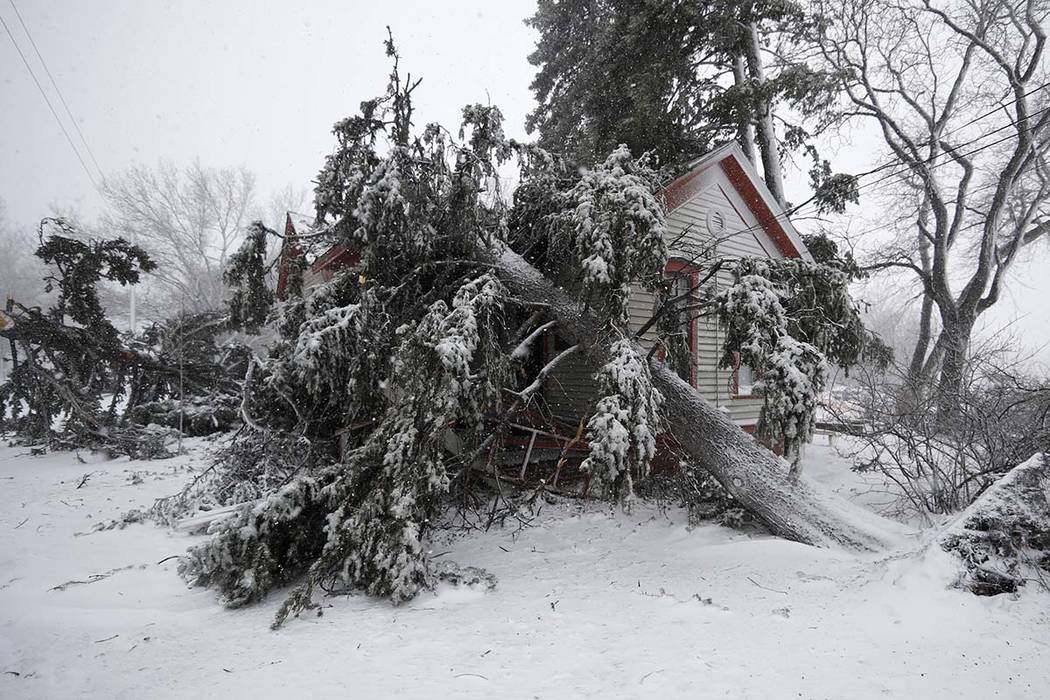The photograph captures a stark and beautiful winterscape dominated by a bright white blanket of deep snow. The scene showcases a modest, almost tiny, white house with red trim around the windows, door, and eaves. This house is nearly fully obscured by an uprooted, large pine tree that has fallen against its side, bringing down some power lines with it. The house appears dark and uninhabited, emphasizing the desolation. Surrounding the fallen pine tree, there are other trees, some standing tall and others seemingly downed in the background, contributing to the scene's sense of chaos from a recent storm. The barren landscape includes several hardwood trees with no leaves to the right and further back, adding to the wintry starkness. The sky is heavily gray, enhancing the scene's cold and somber mood. The whole image is a blend of white snow on the ground, tree trunks, branches, and the house, punctuated by the reddish rust-colored trim of the small, partially buried home.